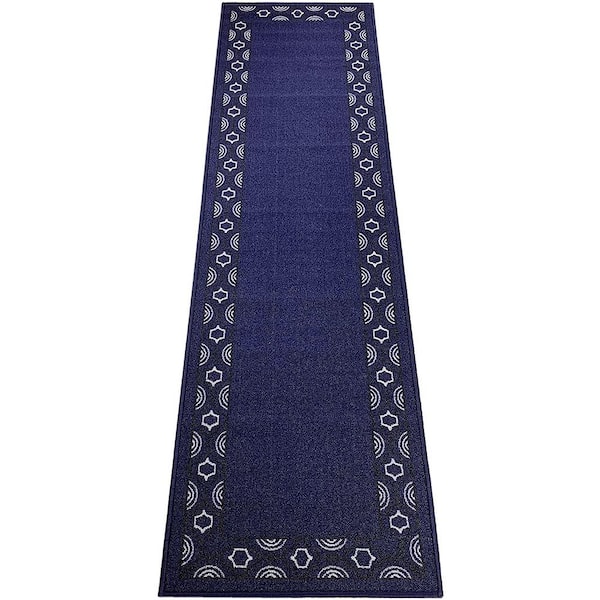The image depicts a long, narrow runner rug in a striking navy blue color, designed to fit perfectly in a hallway. The rug features a low pile, giving it a sleek and modern texture. It is adorned with intricate white trim along its borders, forming a pattern of delicate white shapes and semicircles reminiscent of rainbow designs. These patterns repeat in an orderly fashion along the length of the rug. The overall design is clean and symmetrical, with a central rectangular motif flanked by rows of semicircles. The photograph is set against a plain white background, which emphasizes the rug's elegant and detailed design. The rug’s length is approximately three and a half times its width, underscoring its suitability for elongating narrow spaces.